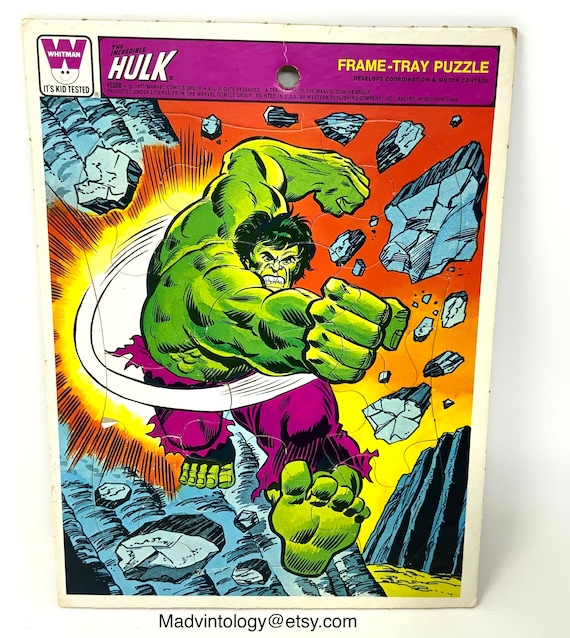This image is the cover of a frame tray puzzle featuring the Incredible Hulk, available for sale on Etsy by Madbentology. The robust, green Hulk is depicted in mid-action, having just punched and shattered a boulder, with his balled-up fists dominating the foreground. His iconic purple pants are torn, and his immense green feet are surrounded by scattered pieces of bluish-gray rock. The background features an intense palette of dark orange and gold, possibly suggesting an explosion or sunburst effect emanating from the impact of his punch. The puzzle, produced by Whitman and labeled as "kid-tested," is bordered by a white frame, approximately the size of an 8.5 by 11-inch sheet. Hulk's snarled face and bared teeth further emphasize the dynamic and powerful scene captured on this puzzle cover.